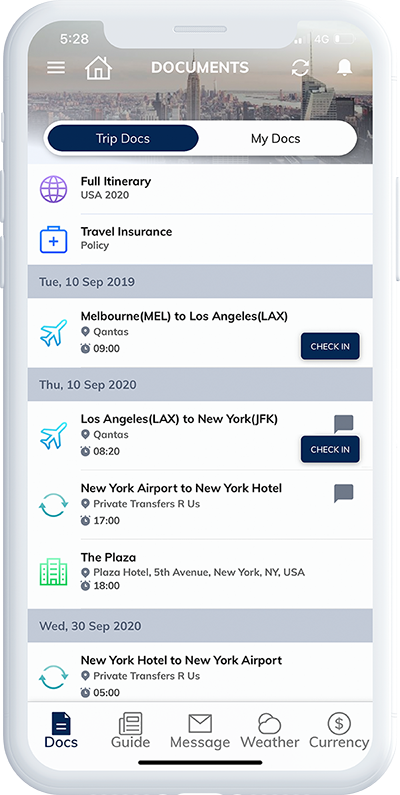This photograph showcases the front screen of a smartphone encased in white or a white case. The top section of the screen displays a cityscape background along with the time, 5:28. Just below this, there is a white bar stretching horizontally across the screen, featuring the tabs "TripDocs" and "MyDocs," with "TripDocs" outlined in blue, indicating it is the selected tab.

Further down, the screen presents an organized itinerary for a trip under the heading "USA 2020," accompanied by a travel insurance policy. A gray line marks the next section which details the first part of the itinerary. On Tuesday, September 10th, 2019, there is a flight from Melbourne to Los Angeles. This section includes an outline of an airplane and a check-in button positioned at the bottom right corner.

The second gray line indicates the next scheduled events for Thursday, September 10th, 2020, with a flight from Los Angeles to New York, followed by a transfer from New York Airport to New York Hotel. A small picture of The Plaza Hotel accompanies this portion of the itinerary. The final section covers the departure on Wednesday, September 30th, 2020, from New York Hotel back to New York Airport, summarizing the end of the trip.